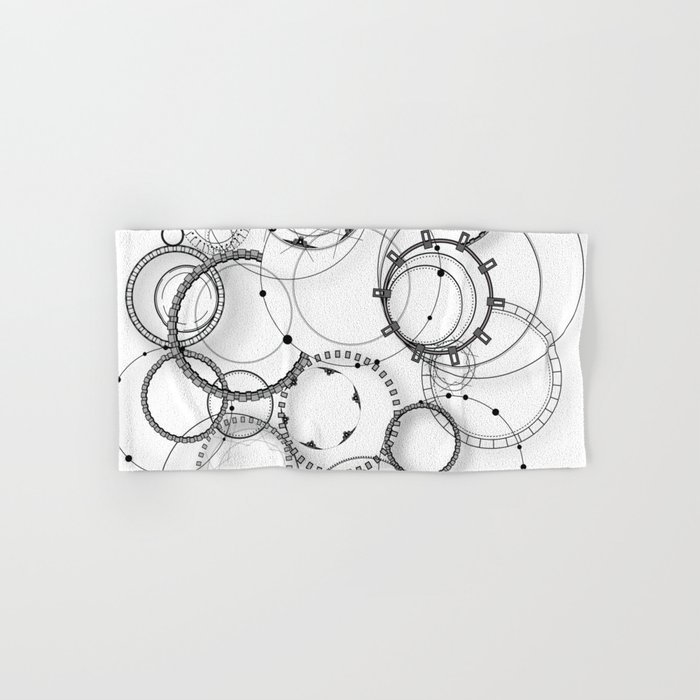A rectangular, featureless gray frame hosts a smaller, computer-generated image resembling a slightly warped white sheet of paper with shadows to the right. This sheet is densely covered with overlapping black-and-white line drawings of circles, each varying in size, thickness, and design. Among the array of circular shapes, some feature cog-like teeth while others have double lines segmented into small squares or beads. The top right section showcases solid black line circles, contrasting with the gray-black, whirlpool-like cluster of rings nearby. One distinct circle, thicker than the rest, has small rectangles with empty centers radiating like clock positions. Other circles include those with two concentric rings connected by radiating lines and some shaded to enhance their curvature. Some feature dots along a thin ring, and the top center circle has a black outline with small, solid black dots. The left side displays designs resembling beaded bracelets, while the bottom section includes circles with dashed lines, creating a rich tapestry of interconnected, diverse circular motifs.